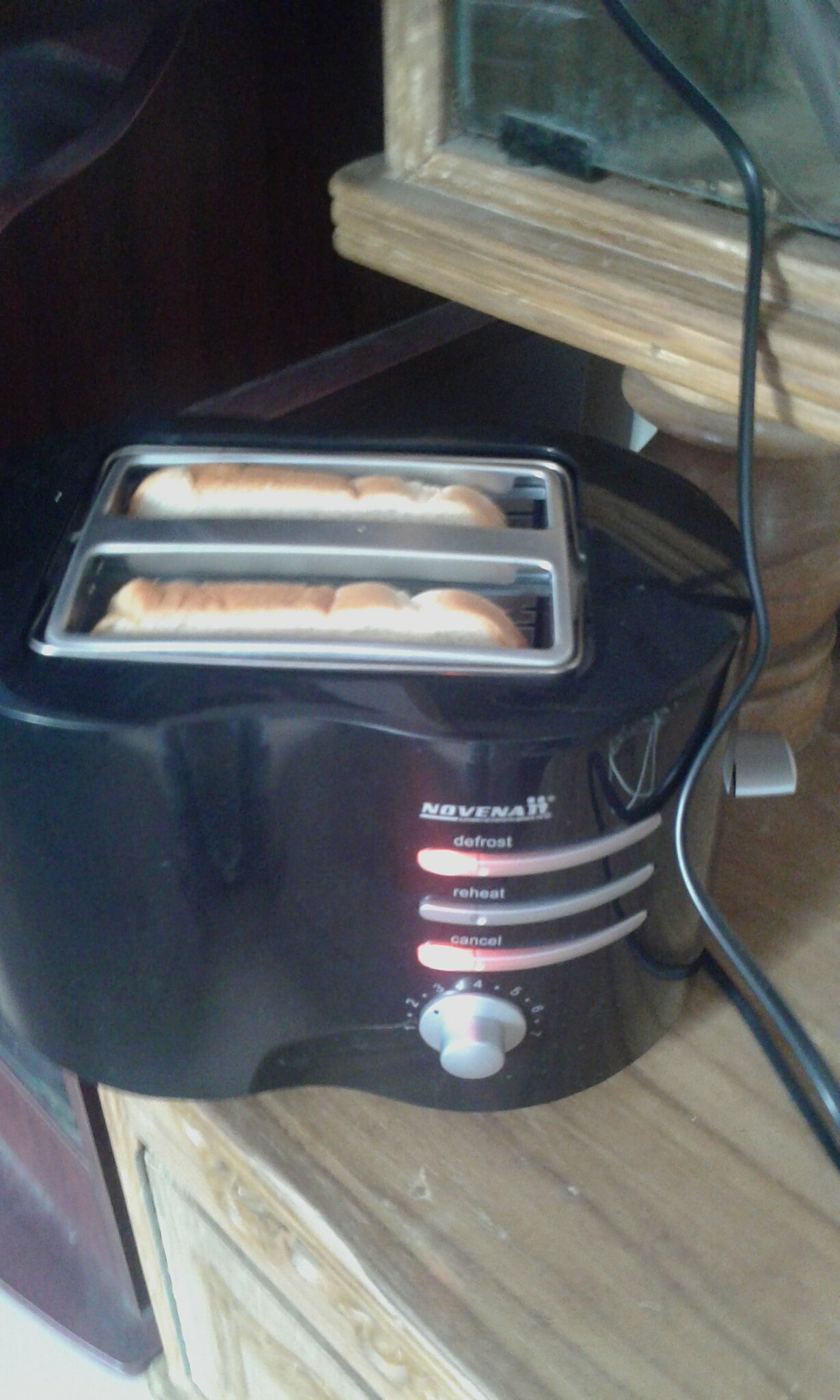The image depicts an amateur photograph of a black plastic toaster branded "Novena," positioned on a wooden surface, likely a kitchen counter or table, adjacent to a glass-paneled storage area or display cabinet. The toaster, which has a capacity for two slices of bread, currently contains two slices of white bread being toasted. The appliance features three light indicators labeled "defrost," "reheat," and "cancel," accompanied by a dial to adjust the toasting intensity from levels 1 to 7. The toaster's black cord is visible, extending across the surface and out of frame. The photograph is somewhat blurry and dark, lacking professional framing or cropping.